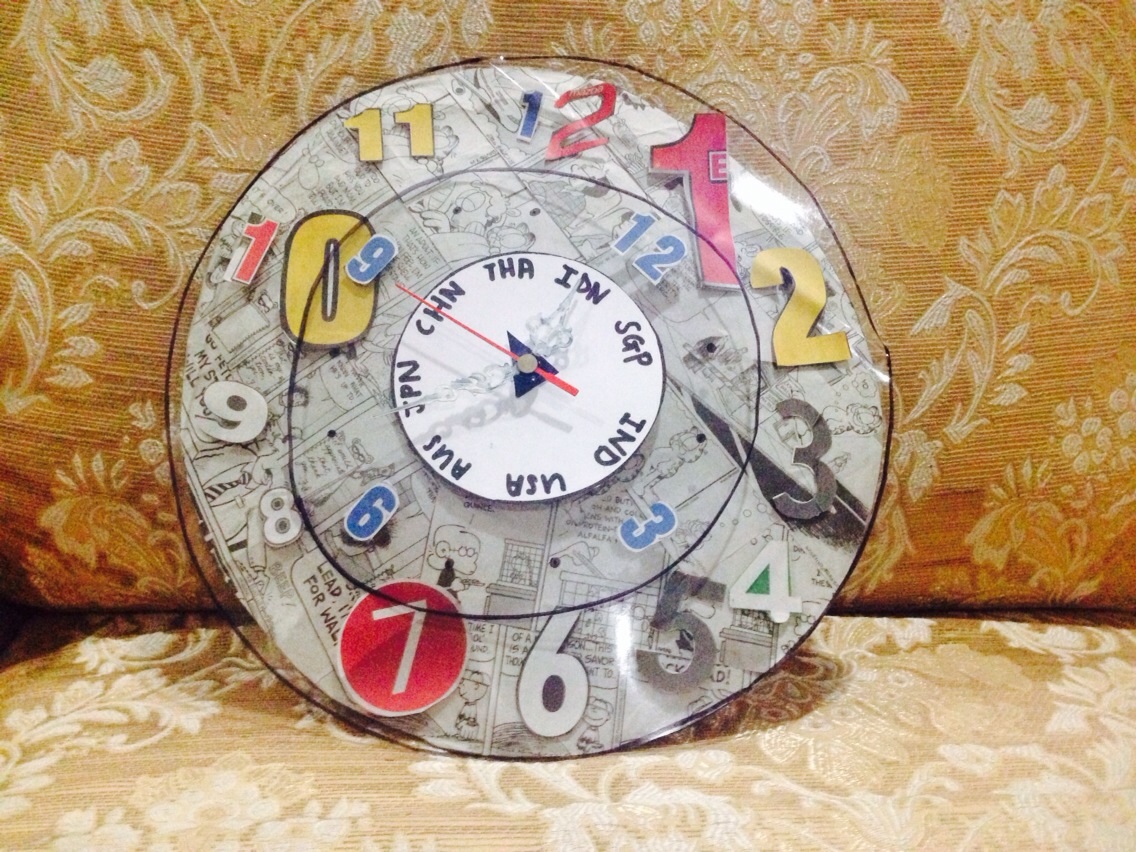This square color snapshot captures an imaginative and whimsical homemade clock. The clock is prominently positioned in the middle of the frame, resting on a gold-embroidered damask or paisley fabric that appears to be part of a sofa or chair. The clock itself is a striking piece of art, featuring a multitude of vibrant and creative details. 

At the outer edge, the clock face is decorated with cutout numbers from various magazines or colored paper, each number differing in size and color, and arranged in the traditional 1 to 12 sequence of a regular clock. On the inner circle, the core clock hands point to the standard positions: 12, 3, 6, and 9. Additionally, this circle is embellished with strips of comic cartoons.

Uniquely, the clock also integrates global elements. It includes a concentric circle within which abbreviations of various countries such as THA (Thailand), IND (India), USA, AUS (Australia), JPN (Japan), and CHN (China) are inscribed. This inner circle is separated by a distinctly drawn black line, creating an organized yet artistic appeal. The clock hands themselves highlight a number, with one notably pointing to 9 in this image.

In summary, this homemade clock is a collage of vivid and eclectic elements, harmonizing everyday materials and artistic creativity, all set against a textured gold fabric backdrop.